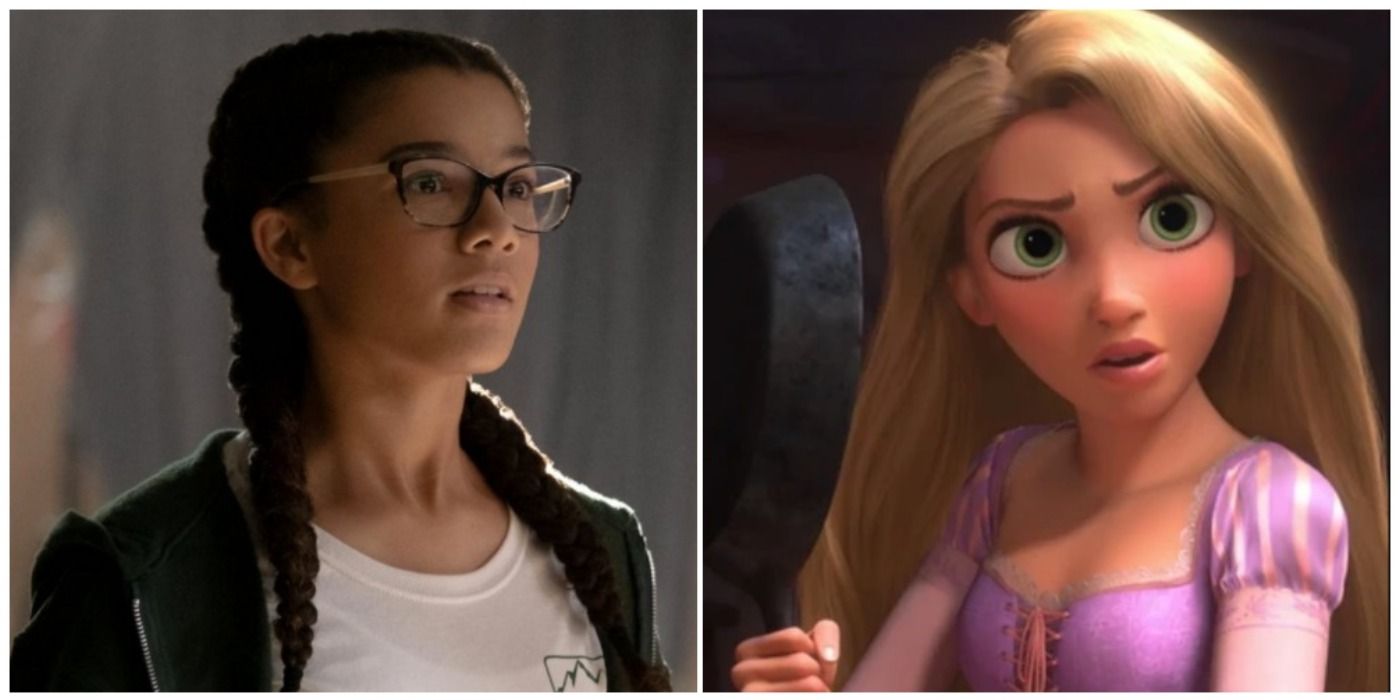The image is a rectangular collage of two square photographs side-by-side. On the left is a photograph of a surprised teenage girl with dark hair styled in two braids, wearing black glasses, a white T-shirt, and a black jacket. Her background is gray and blurred, and she is staring intently to her right. On the right is an animated illustration of a fairytale princess with long blonde hair, large green eyes, and furrowed brows, dressed in a purple outfit. She also looks surprised and is holding something ambiguous in her hand. The detailed expressions in both images convey a sense of shared astonishment and curiosity towards each other.